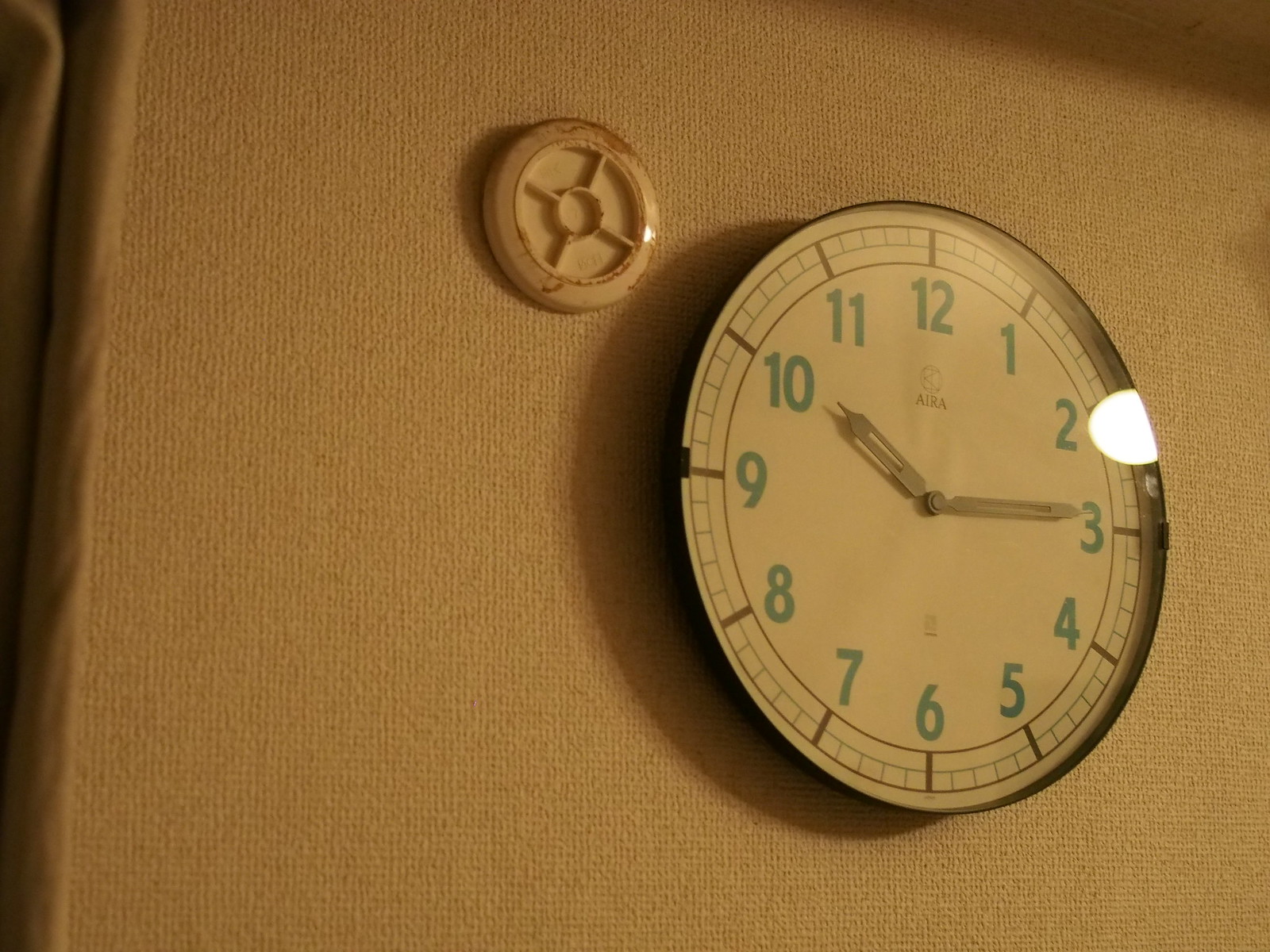This close-up photograph captures a clock mounted on a textured tan wall. The clock features a white face with blue numbers marking the hours from 1 to 12, starting at the top center. Black hashes along the periphery indicate the minutes, with white hashes in between them. The time on the clock is set to approximately 10:14, as the silver hour hand points slightly past the 10 and the silver minute hand points at the 3. The clock also has a distinctive reflection of a white light on its right side. At the center of the clock face, the word "A-I-R-A" is inscribed in black letters. Near the clock, a round object resembling the base of a smoke detector, featuring a brown color with brown and tan splotches covered by a clear plastic casing, is also mounted on the wall.